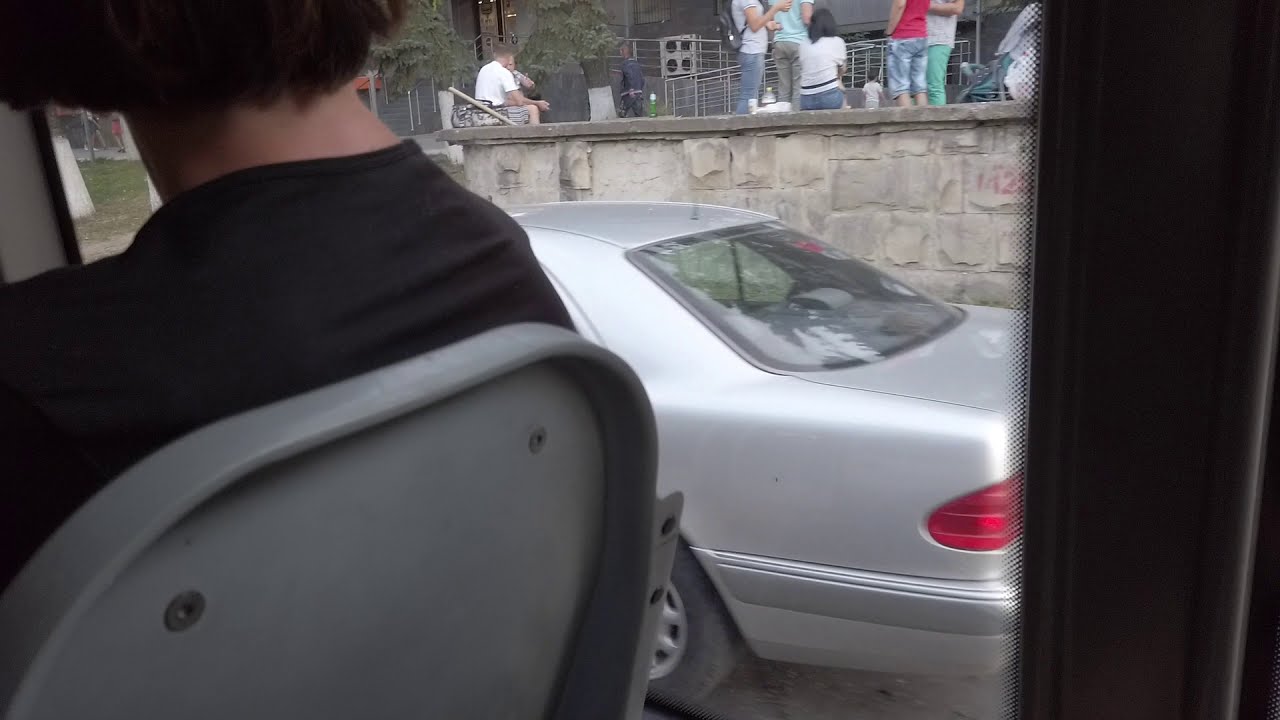The image depicts the upper back, shoulders, neck, and head of a person with dark brown hair, wearing a black shirt, sitting in a hard-backed gray metal chair. The viewpoint is from inside what appears to be a bus, and the person is looking out a window. Through the glass, there is a static, gray sedan car just outside. Beyond the car lies a stone wall next to which a group of people are standing or sitting, engaged in various activities that suggest a setting like a park or an open patio area. Some people are sitting in a relaxed manner, possibly socializing, while others are standing in small clusters. The background includes trees and a box with four black circles, possibly a speaker, indicating an area where people might gather for events or casual meet-ups. The scene is detailed with the presence of railings and tubing, adding to the urban, public space feel of the surroundings.